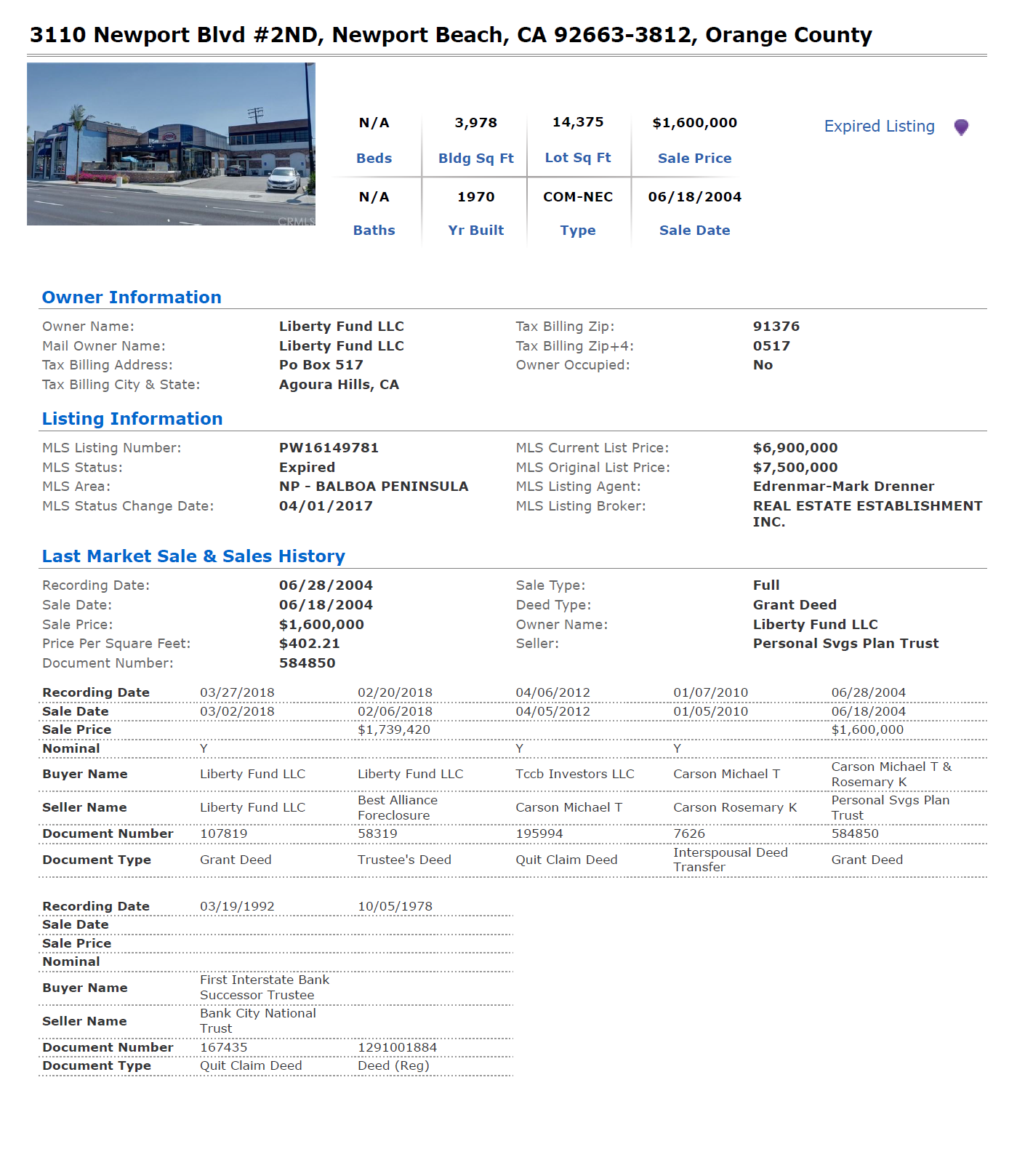This commercial real estate listing is located at 3110 Newport Boulevard, Unit 2ND, Newport Beach, California, in Orange County. The property is owned by Liberty Fund LLC from Agoura Hills. Listed through Real Estate Establishment Inc., the current asking price is $6,900,000, down from the original list price of $7,500,000. The commercial building, which was built in 1970, spans 3,978 square feet and sits on a lot approximately 14,000 square feet in size. The property is zoned for commercial use, and although it features no bedrooms or bathrooms, the detailed listing information is available for serious investors.